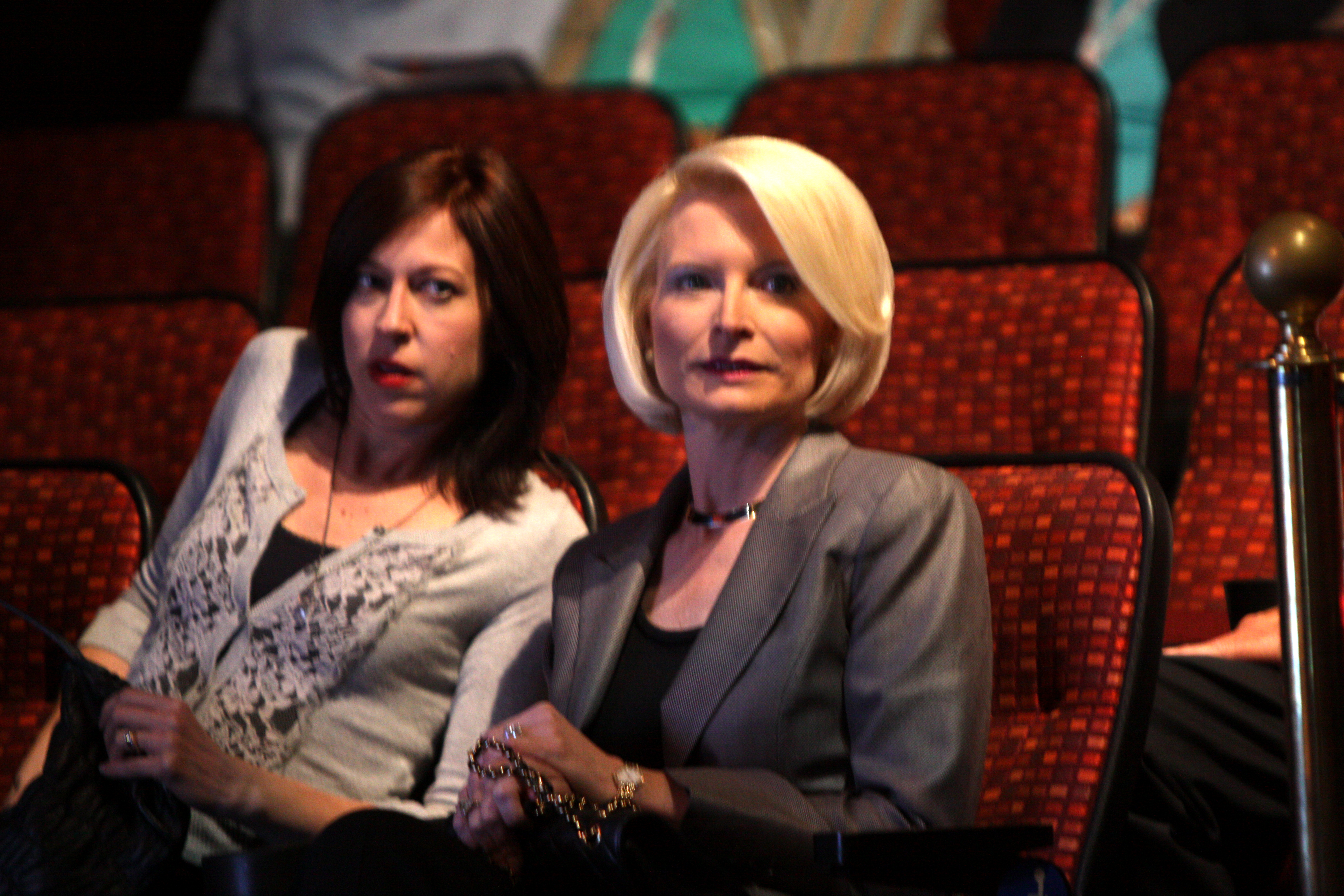In the photograph, two women are seated in the first row of a modern cinema, characterized by multiple rows of plush red chairs. The woman on the left, appearing to be in her late 40s or early 50s, has short blonde hair and wears a gray jacket over a black undershirt. She exudes a business-casual vibe. To her right, a slightly chubby woman with reddish-brown hair, styled straight and cascading over her ears, leans in her direction. She is dressed in a white cardigan over a black top, accentuated with a necklace and red lipstick. Both women gaze intently off to the right side of the image, seemingly captivated by something beyond the frame. Although the first three rows are completely empty, dimly-lit figures can be discerned in the fourth row. The cinema's aisles and lighting suggest an intermission or pre-show ambiance, adding a sense of anticipation and curiosity to the scene.